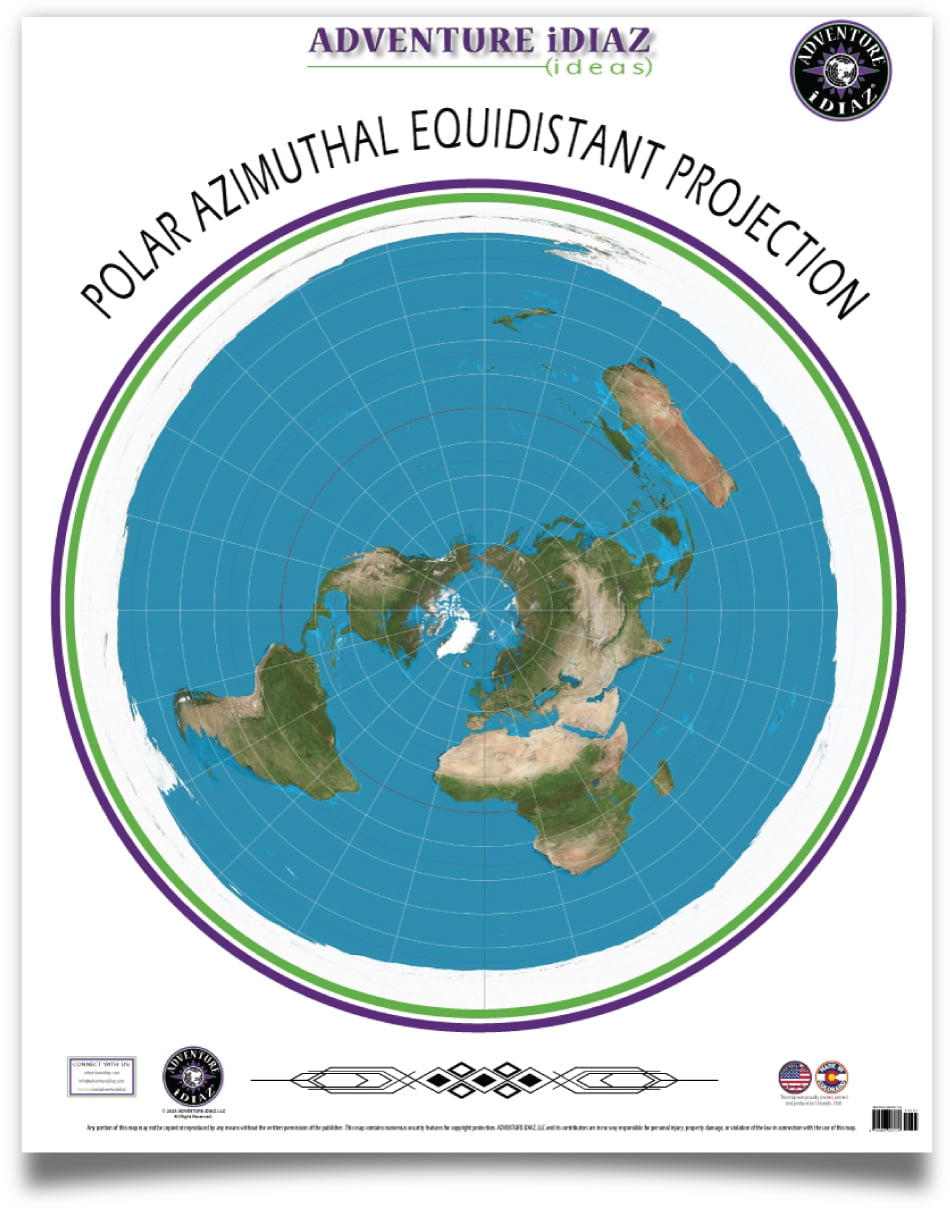The image showcases the cover of a book with a primarily white background. At the center, there is an artistically rendered globe, viewed from above, featuring imperfect lines and bordered in brown. The top of the cover displays the text "Adventure Ideas," with "Polar Azimuthal Equidistant Projection" positioned directly beneath it. In the lower right corner, a small circular emblem with a fragment of the American flag is visible, alongside a black scan code. The lower left corner features a black circular logo containing the words "Adventure Ideas" in white text.